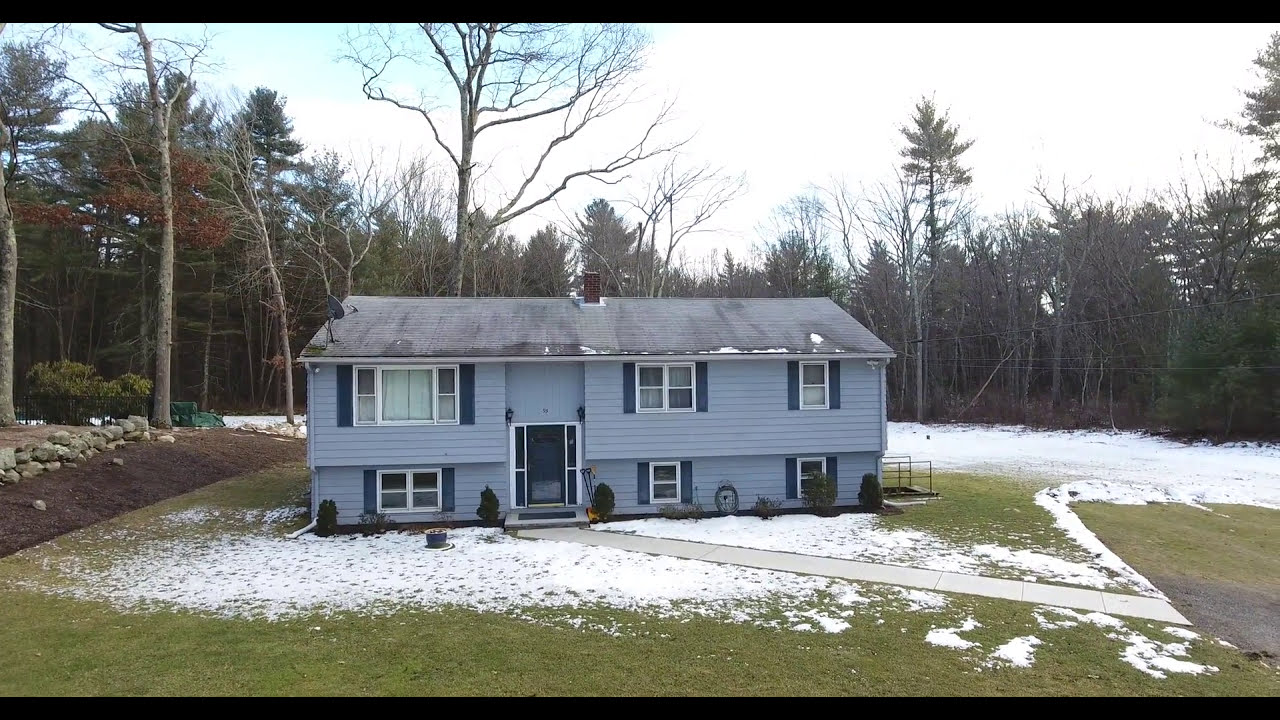This image showcases a light blue, two-story house with an older, east coast architectural style. The house has an arched roof with black tiles marred by water stains, and a chimney protruding from the middle, accented by a white base. A satellite dish is affixed to the bottom left corner of the roof. The exterior features panel siding, with siding running horizontally. 

The top floor displays three windows: the leftmost window has curtains hanging in the middle and consists of a larger central window flanked by two smaller windows, all framed in white. The central window on this floor has four panels and is bordered by blue rectangles, while the rightmost window is a two-paneled design. 

The ground floor includes a four-paneled window on the far left, followed by the front door with a screen, another two-paneled window, and a final two-paneled window partially obscured by a green bush. A grassy front yard, with patches of snow interspersed, transitions into a long cement pathway that leads from the front door to the right side, where parking seems to be located. 

Behind the house lies more snow-covered ground and a dense, tall row of trees, some leafless and some partially leafed, adding to the wintry atmosphere. The sky overhead is mostly a hazy white, with a hint of light blue in the upper left corner, contributing to the overall serene, chilly mood of the scene.